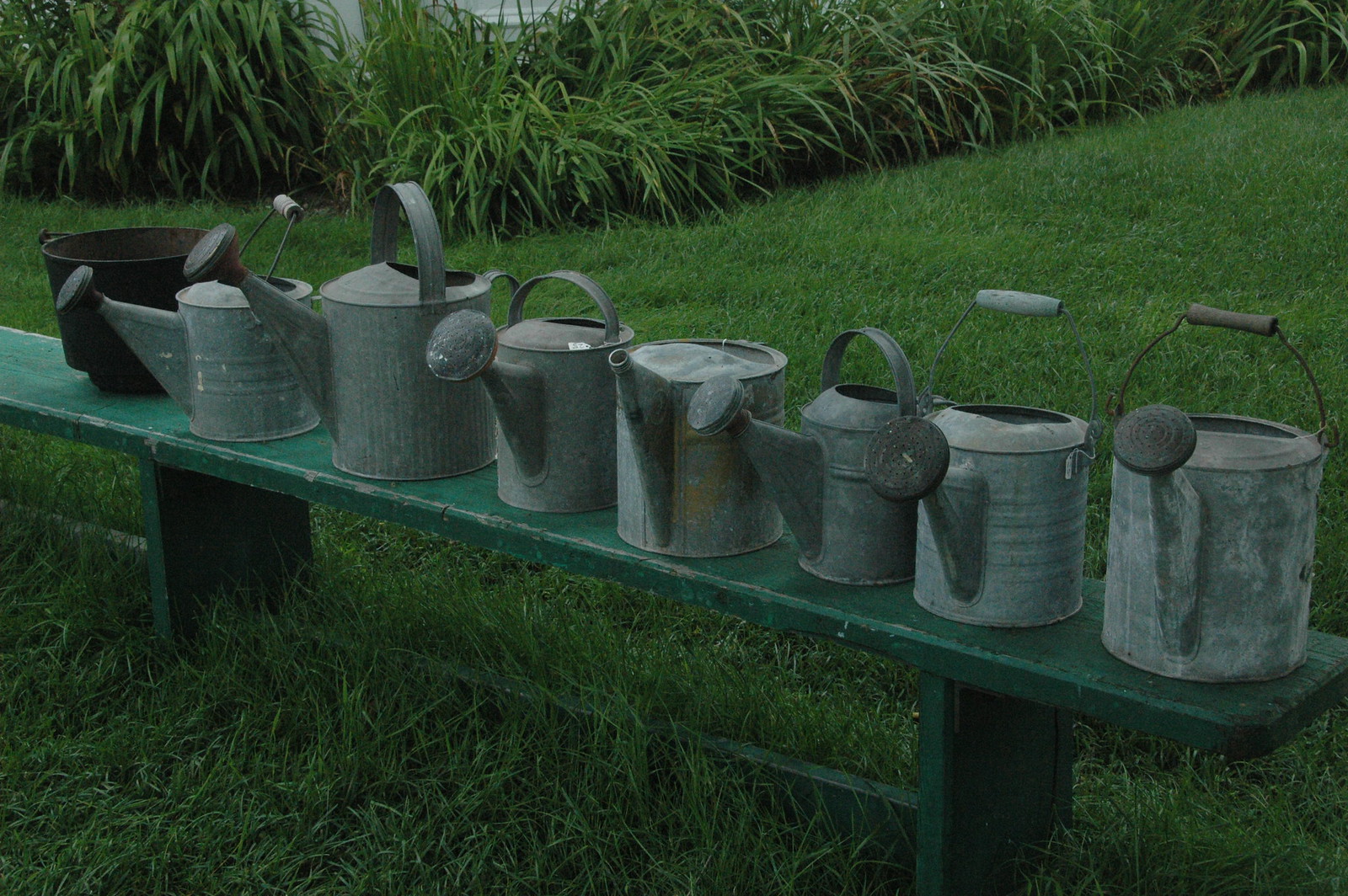The photograph captures an outdoor scene featuring an old green wooden bench set against a lush green grass field. Adorning the bench are seven vintage watering cans, predominantly made of galvanized tin or steel, exhibiting wear with visible scratches, splotches, and patches of rust. These watering cans vary in shape and size, with some having large spigots and others smaller ones. Additionally, each has distinct handles, from thin to large, enhancing their aged and well-used appearance. On the far end of the bench sits a dark brown bucket-like structure. In the background, there are verdant plants with long, drooping leaves and a glimpse of a white structure, likely a house, adding depth to the setting.